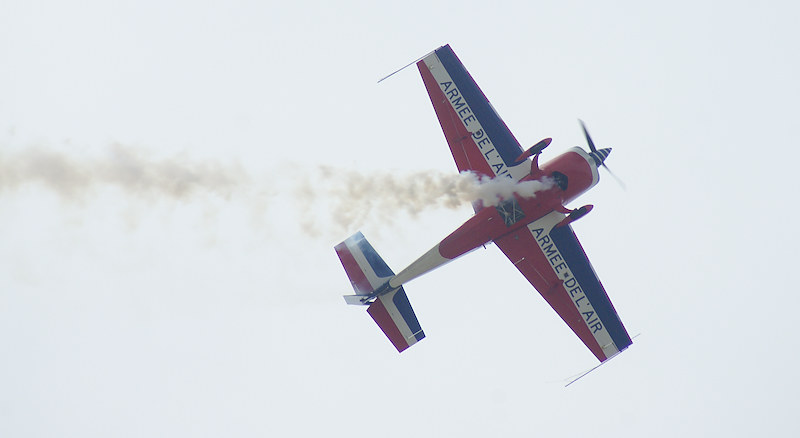This image captures a vibrant stunt plane in mid-flight, angled from the bottom left to the upper right, with a trail of gray smoke streaming horizontally to the left. The aircraft's body is predominantly red with a white section near the tail. Both the wings and the tail are adorned with blue, white, and red stripes. The wings showcase inscriptions in blue on the white stripes, reading "Armée de l'Air." From beneath, you can see a spinning propeller featuring a blue and white striped tip. Just behind the propeller, a silver ring is visible, adding contrast to the design. The plane appears to be a two-seater, with two cockpits, and the detailed color scheme includes blue on the top sections of the wings, white in the center, and red on the bottom. The image beautifully illustrates the dynamic motion of the stunt plane against the sky.